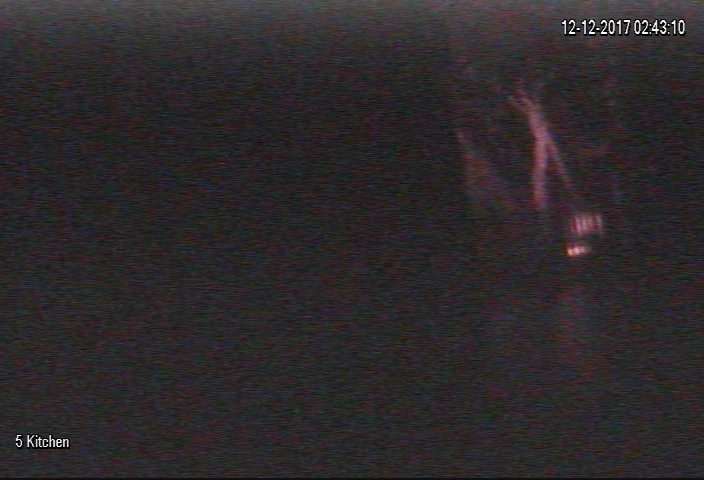This nighttime image is quite blurry, making it challenging to discern specific details. A timestamp in the top-right corner reads "12-12-2017 02:43:10 AM," indicating the photo was taken on December 12, 2017, at 2:43 and 10 seconds in the morning. The bottom left corner is marked with "5 Kitchen," suggesting that the image was captured by the fifth security camera installed in a kitchen area. A noticeable greenish glare appears prominently in the image, adding to the difficulty of making out any clear features.